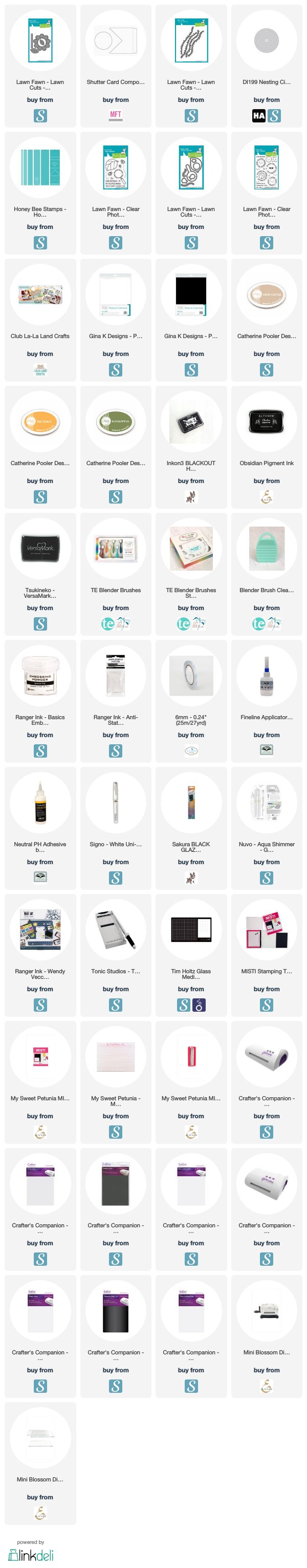The displayed image is an amalgamation of numerous small pictures, predominantly showcasing various crafting supplies and equipment, specifically from the Lawn Fawn Lawn Cuts series. At the forefront, there are intricate stencil designs intended for lawn-related projects, including a gray flower with seeds labeled as part of the Lawn Fawn Lawn Cuts collection, available for purchase. Adjacent, there is information regarding a Shutter Card composition available from MFT, also part of the Lawn Fawn series.

The layout transitions from lawn equipment and accessories, encompassing items like grass seeds and other related products, to an assortment of craft supplies. These include nesting stamps from Lawn Fawn's clear selection, among other miscellaneous tools and materials essential for crafting. At the bottom, the image indicates that the compilation is powered by Link Deli.

Further down, the collection diversifies significantly, featuring products from various crafting brands such as Club La-La Land Crafts, Gina K Designs (in both black and white), Catherine Pooler Designs (highlighting shades like sandcastle, orange, and green), and blackout ink. There's also mention of different applicators. Each small picture meticulously presents these products, reflecting a wide array of crafting essentials spanning from inks in varied colors to precision application tools, portraying a comprehensive resource for craft enthusiasts.